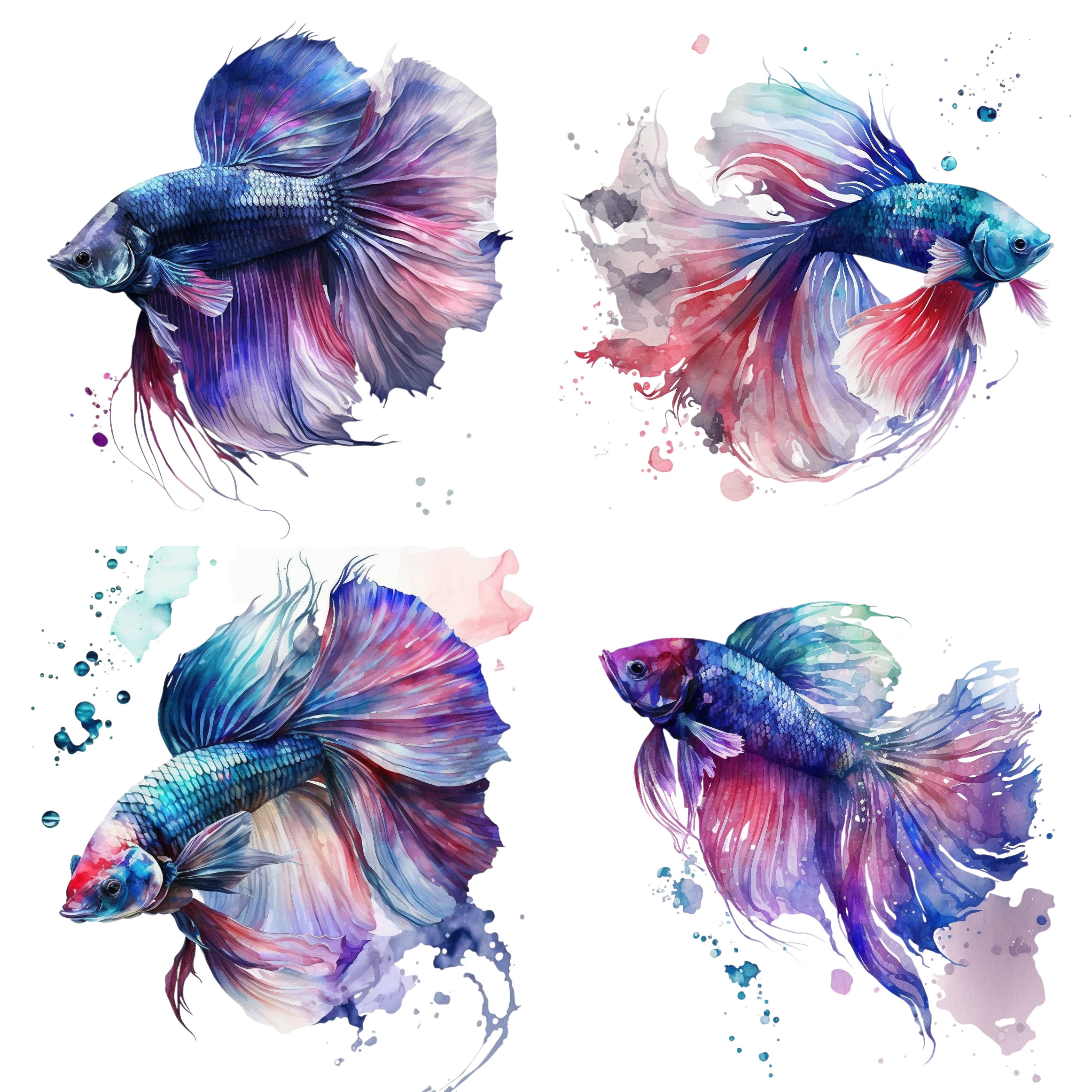The image depicts a detailed painting of four colorful betta fish set against a white background, creating a striking visual effect. Each fish exhibits majestic and ethereal qualities with their large, fanned-out fins and tails that almost resemble wings. The fish appear to be swimming gracefully, despite the absence of visible water. In the top left, a predominantly dark blue betta fish with reddish, white, and bluish fins looks to the left. The top right features a slimmer fish, primarily green with whitish and red fins, gazing to the right. Below them, on the bottom right, a fish with a red head, blue body, and similarly elaborate fins faces left. To the left of this one, another betta fish with a light blue face and a red-tinted head also looks left, adorned with its beautifully spread-out fins. The vibrant colors of purples, blues, reds, and greens create a harmonious display, emphasizing the intricate and colorful design of each fish.